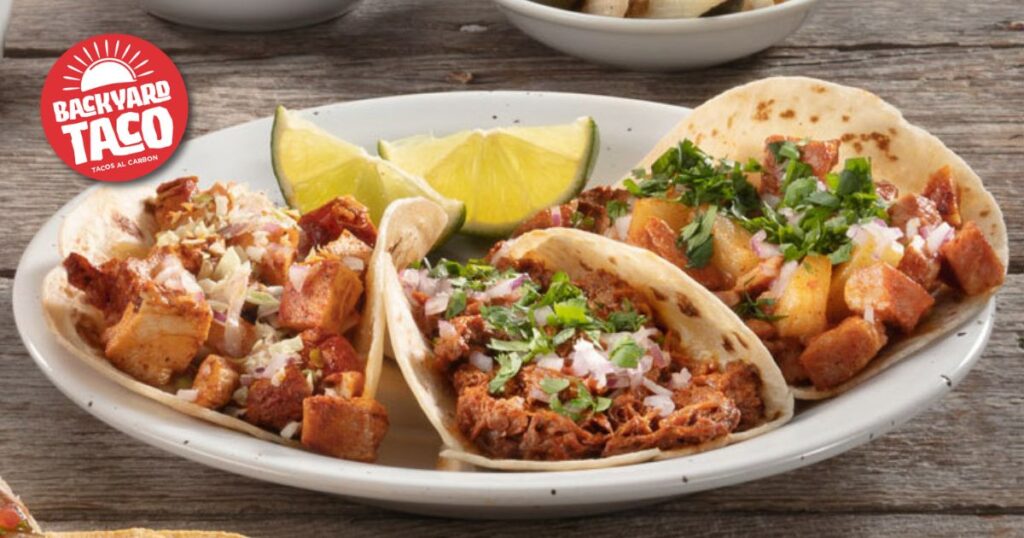The image showcases a white plate with minor imperfections, set on a brown and light tan wooden picnic table, holding a delightful arrangement of three open tacos. The tacos are generously filled with beef, accompanied by onions and bits of lettuce, with hints of cilantro and cheese. Two lime wedges are placed behind the tacos, adding a splash of vibrant green to the composition. In the top left corner, the plate also features a red circular logo with white text that reads 'Backyard Tacos' and an illustration of a sunset with radiant lines, indicating the likely setting of a casual outdoor meal or a picnic. In the background, two bowls add to the scene, enhancing the inviting and rustic ambiance.